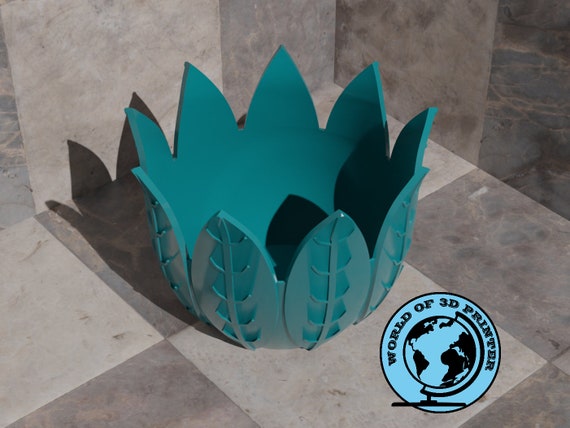A color photograph showcases a 3D-printed turquoise object that combines the aesthetics of a vase and an ashtray. It is designed with petal-like shapes and leaf patterns, which feature leaf veins branching out down the middle. This intricate object is placed on a checkerboard background, comprised of light gray and darker gray marble tiles, with the same pattern extending upwards on the adjacent wall, resembling the inside of a shower. The light source, positioned from the top right, casts a shadow of the 3D-printed creation towards the left. A logo positioned in the lower right corner of the photo features a light blue circle containing a partial globe illustration in black. Surrounding this globe is the text “World of 3D Printer” in black, completing the scene.